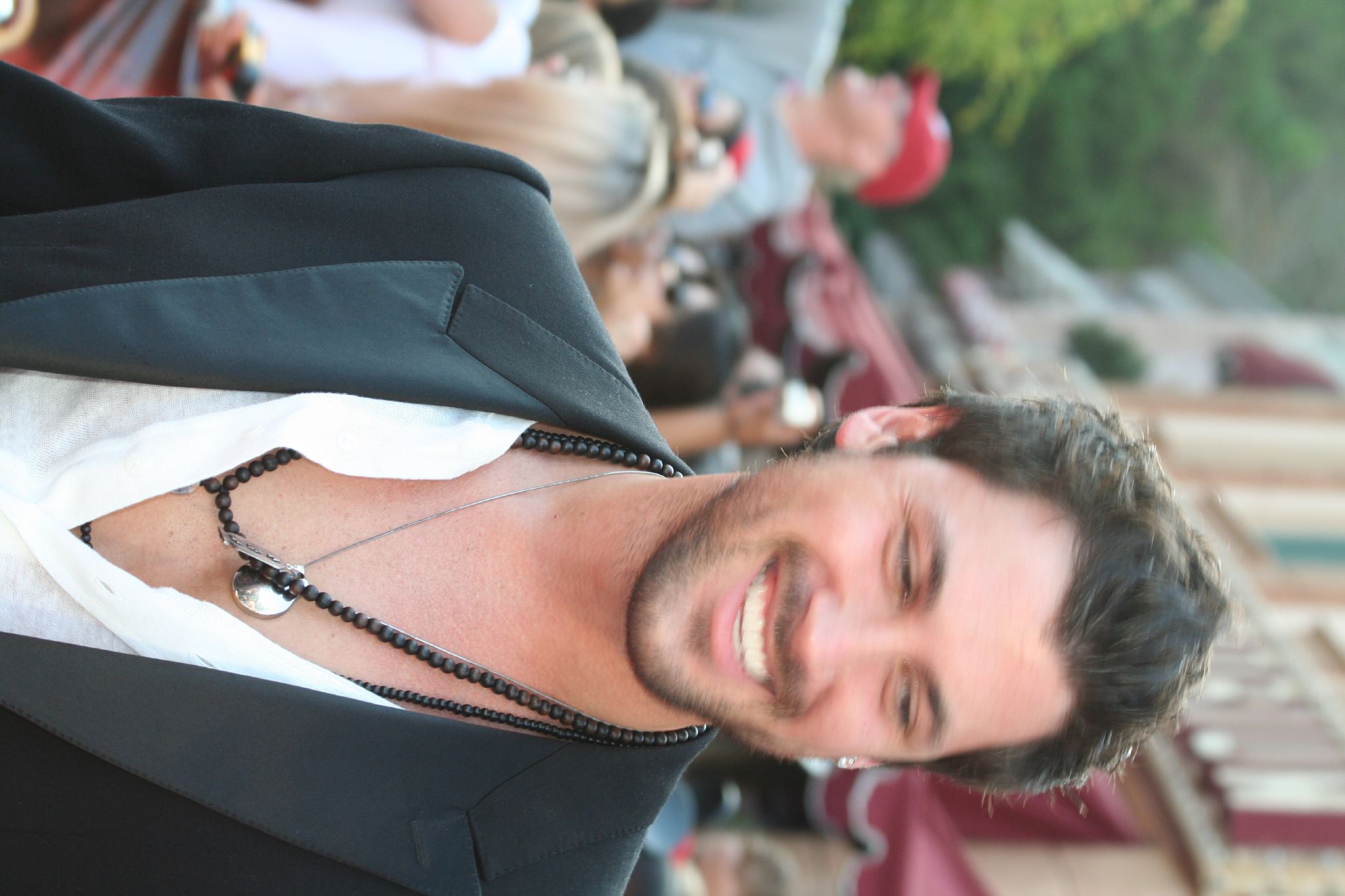The image depicts a slightly blurry, rotated photograph of a smiling, middle-aged Caucasian man with medium-length brown hair that is combed and slicked back. He wears a white shirt, unbuttoned, with a thick-collared black jacket. Around his neck, he sports various jewelry: a black beaded necklace with two strands of beads—one larger and one smaller—and a thin silver chain with a silver medallion. His thin mustache and beard contribute to his cheerful expression, accentuated with crow's feet around his eyes. A small earring adorns his right ear. The background, which is out of focus, suggests an outdoor setting with people, buildings, and trees, indicating he might be at an event. The image cuts off at the man's chest, emphasizing his upper body and attire.